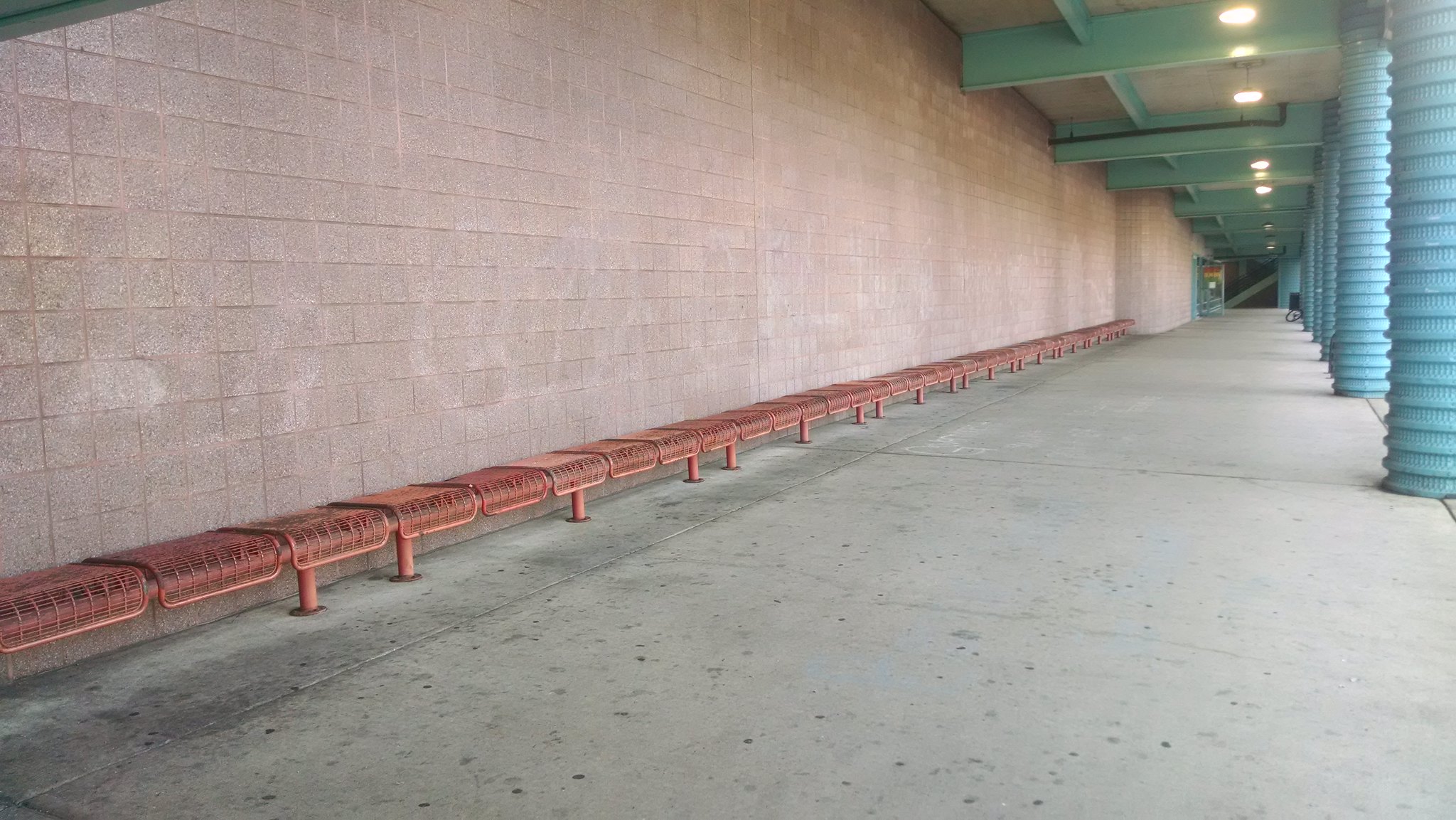The photograph depicts a long, outdoor breezeway or concourse area that appears to be part of an educational institution. The left side of the image features a long, square-bricked wall in a light pinkish-red tone. At the base of this wall, a steel bench with individual seating sections is bolted to the concrete floor. The bench is colored reddish-pink and has round pillars extending halfway into the distance, sprayed in red. The ground is made of cement, and the breezeway is covered at the top with a cement ceiling featuring recessed lighting. Along the right side of the image, perpendicular to the wall, are vibrant turquoise-blue corrugated pillars that resemble the striated sections of bendy straws. Although the sky is not visible, daylight illuminates the pathway from the right. In the distance at the far end of this long walkway, stairs are visible, leading upward, suggesting a continuation of the structure beyond the frame.